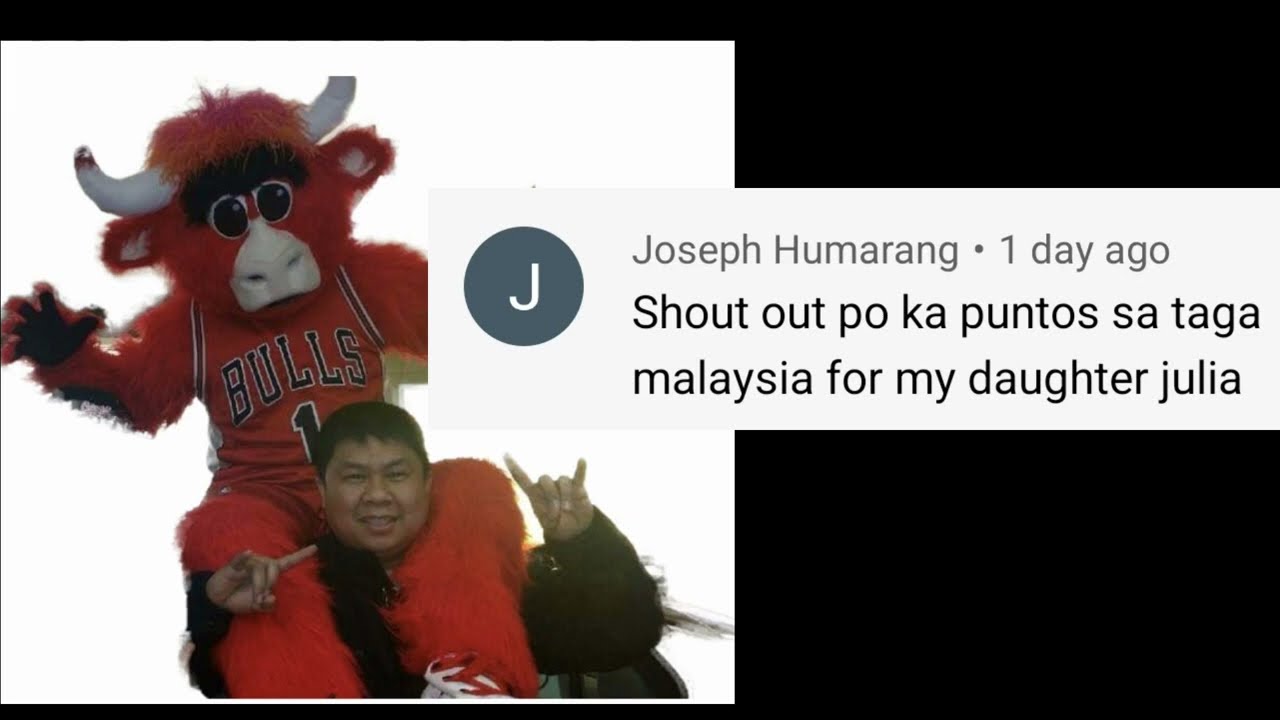In this vibrant, energetic photograph, we see an Asian man wearing a black sweatshirt posing with a lively expression. His left hand is raised, gesturing a devil sign with his fingers while his right hand points towards the sign. Perched on his shoulders is the Chicago Bulls mascot, an animated bull adorned in a vivid, furry red costume complete with white horns and a mask. The mascot sports a Chicago Bulls jersey emblazoned with the number one and the word "BULLS" across the front. Cutting diagonally across the image is a white stripe bearing text. In this stripe, inside a dark blue circle with a white letter 'J,' the comment reads: "Joseph Humaring, one day ago, shout out Pokah Puntisataga Malaysia for my daughter Julia." This detail indicates a proud parental shoutout, likely shared on social media.